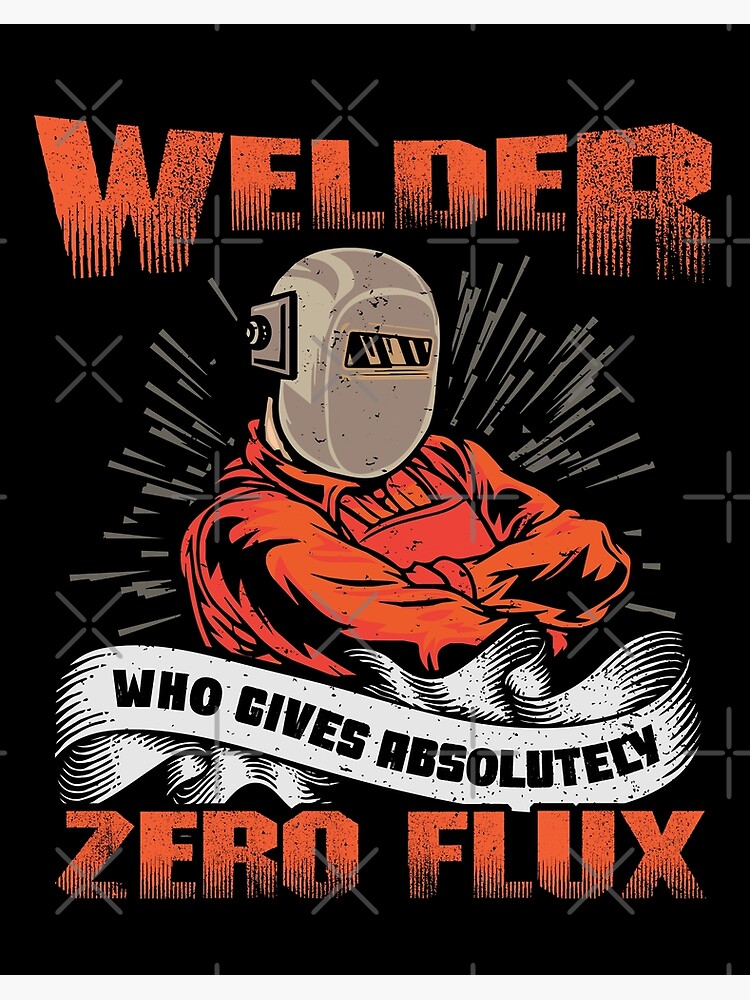The image features a stylized animation set against a black background. Dominating the top of the image are the bold, orange capitalized letters spelling "WELDER." Below this text stands a figure clad in an orange long-sleeve shirt and a matching apron, with their arms crossed confidently. The person’s face is entirely obscured by a large, rounded gray welding helmet, complete with a rectangular view screen. Centered on the image, just below the welder's folded arms, is a white ribbon that displays the phrase "WHO GIVES ABSOLUTELY." Directly beneath this, in orange, capitalized letters matching the header, are the words "ZERO FLUX," a clever play on the phrase. The overall design highlights the words and the figure’s assertive stance, employing a color scheme of orange, black, white, and gray.